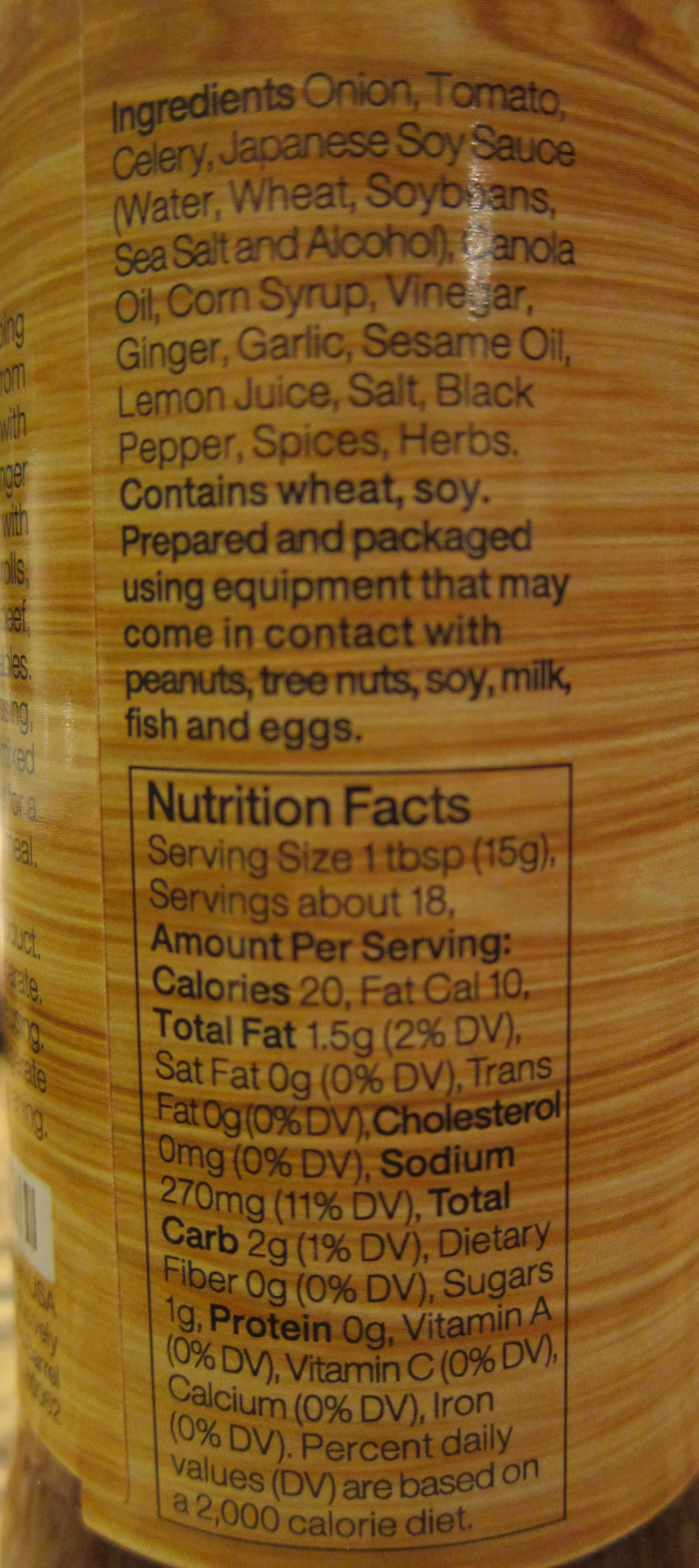This color photo on the side of a bottle or can showcases ingredients and nutritional facts against a wooden-patterned background that resembles bamboo. The text is in black. The ingredient list reads: onion, tomato, celery, Japanese soy sauce, water, wheat, soybeans, sea salt, alcohol, canola oil, corn syrup, vinegar, ginger, garlic, sesame oil, lemon juice, salt, black pepper, spices, and herbs. It also notes that the product contains wheat and soy, and is prepared and packaged using equipment that may come into contact with peanuts, tree nuts, soy, milk, fish, and eggs. 

Below the ingredient list, enclosed in a thin black rectangle, are the nutritional facts. The serving size is one teaspoon (15 grams), with approximately 18 servings per container. Each serving contains 20 calories, with 10 calories from fat. Total fat content is 1.5 grams (2% DV), which includes 0 grams of saturated fat and trans fat (0% DV each). Cholesterol is 0% DV. Sodium varies from 20 to 70 milligrams (11% DV). Total carbohydrates are 2 grams (1% DV), including 1 gram of sugar and 0 grams of dietary fiber and protein. Vitamin A, Vitamin C, calcium, and iron are all 0% DV, based on a 2,000 calorie diet.